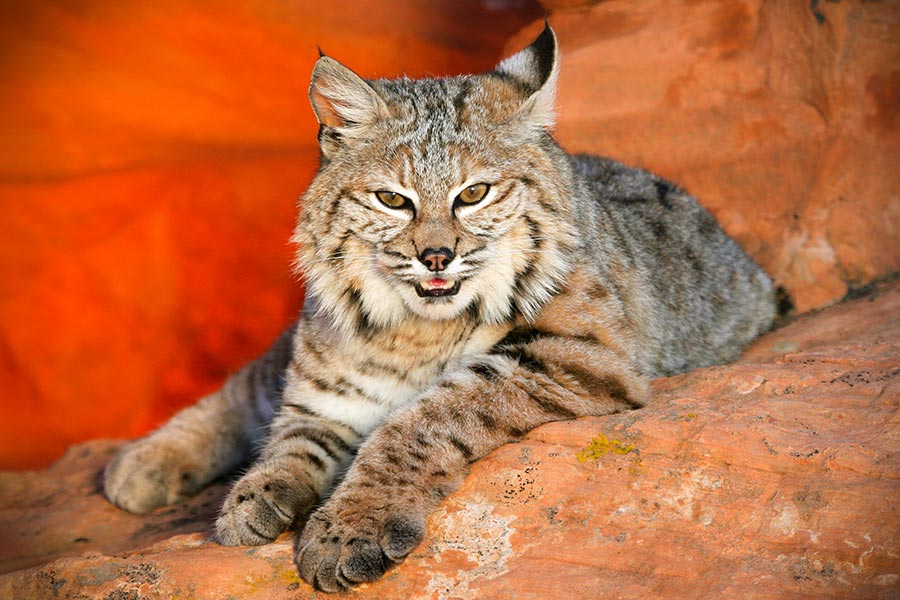This is a horizontal rectangular photograph of a cat, possibly a bobcat or a lynx, featuring striking details that highlight its wild and majestic nature. The cat is reclining on a comforter that superficially resembles an orange boulder, making it ambiguous whether this is an indoor setting or a natural rock formation. Its fur is a mix of brown, white, and gray, with noticeable black stripes. The cat's face is oriented towards the camera with slanted, yellow eyes that give an intense, piercing look. One ear is turned sideways while the other faces forward, adding to its alert expression. The cat's mouth is slightly open, revealing its teeth and tongue, and there is white fur around its chin and neck that almost gives the appearance of a smile. Its whiskers extend straight to the sides of its nose. The front paws are brown and appear tucked under its head, while a third leg is visible in the background. The bright, neon-like orange shade of the surrounding stone, which appears almost to glow, enhances the dramatic and wild aura of the scene.